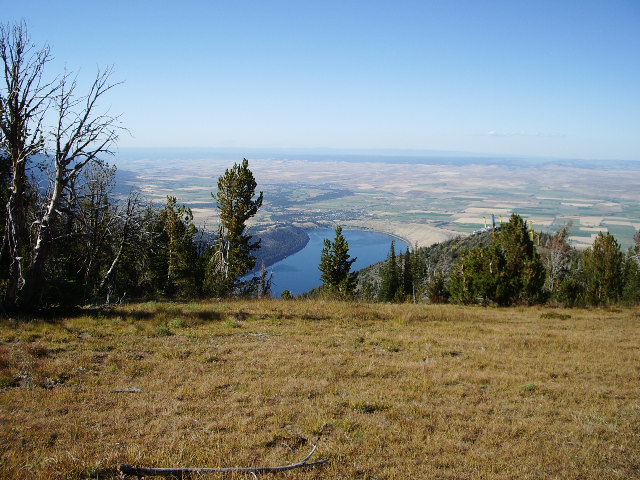This captivating photograph, taken from a high vantage point atop a hill or mountain, offers a stunning panorama of a vibrant natural landscape seamlessly melding into a distant urban setting. In the foreground, lush green grass and a prominent branch frame the scene, leading the eye towards a dense cluster of trees and bushes. As the view extends further, a meandering river or stream gracefully curves through the landscape, serving as a natural divide between the verdant expanse and a distant town or city that sits along both of its banks. On the horizon, where earth meets sky, the hint of a larger body of water is just perceptible beyond the distant land. The sky above is clear and crisp, painted a brilliant blue, accented only by a faint smattering of clouds in the far back right corner of the image. The color palette is dominated by the rich greens and browns of the vegetation, intertwined with the serene blues of the water and sky, creating a harmonious and tranquil vista. The photograph, devoid of any human presence or text, beautifully encapsulates the peaceful coexistence of nature and civilization.